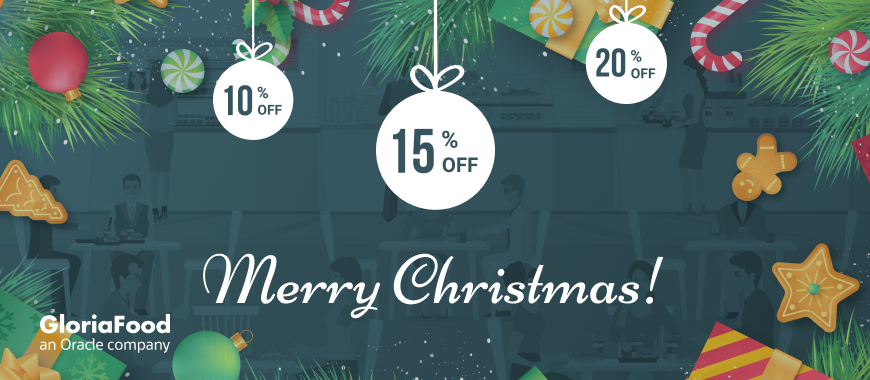A festive and inviting landing page is adorned with a variety of Christmas-themed decorations, perfect for indulging in the holiday spirit. On the left side, a cluster of evergreen trees sets a
seasonal tone. An eye-catching red ornament with a brass or gold cap occupies this section as well, its design completed by a smaller semicircle at the top. Nearby, a Christmas cookie shaped like an evergreen tree stands out against its orange background. The tree is intricately decorated with white icing.

Toward the lower left, more evergreen branches—with deep green hues—grace the page. A dark green present covered in snowflake patterns, both dark and light green, also draws attention. This gift is wrapped with a gold ribbon adorned with the bold white text "Gloria Foods," followed by "G-L-O-R-I-A Food" in regular white text, identifying it as an oracle company.

Central to the design, the words "Merry Christmas" are written in bold, cursive white text, providing the page's festive greeting. Mints are scattered throughout the top background: one is green with a light green center and white spirals, another is orange with white spirals, and yet another is a traditional red and white striped candy cane. A second candy cane is found on the right-hand side along with a classic red and white mint.

Among this candy-coated flurry is a vibrant gingerbread man in orange-brown tones. A star with an intricate design and a green center also stands out, adding a touch of elegance. A red present with yellow stripes and a gold bow sits nestled on the lower right-hand side.

Cascading down the page are small, bulb-like ornaments featuring text. One green bulb offers "10 percent off," another announces "15 percent off," and a final bulb presents "20 percent off," adding a layer of festive excitement and incentives for the visitors.